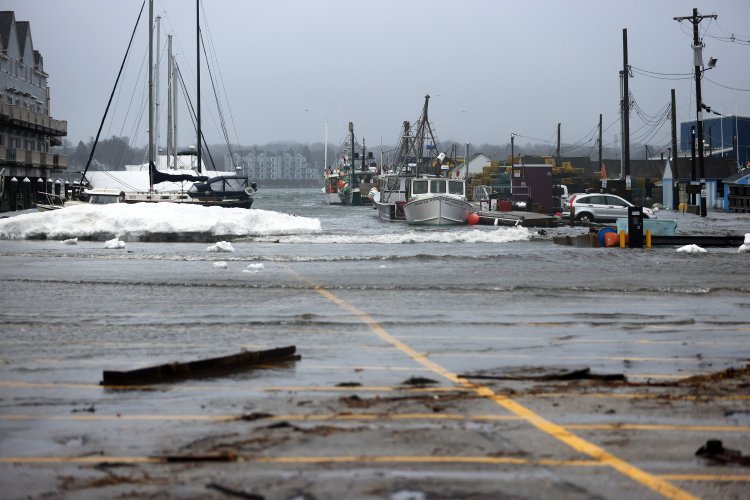The image captures a dramatic scene during what appears to be a storm or natural disaster. A once-functional coastal parking lot is now engulfed by violent, crashing waves, flooding the area and leaving it littered with debris. The ground is a blacktop covered with yellow parking lines, now barely visible under the encroaching water. Off to the right, a gray SUV is parked near a cluster of flagpoles and a dock, emphasizing the human aspect of this disrupted landscape. The dock area extends further to the left, where grayish-blue houses line up beside an array of fishing boats, characterized by their tall masts and cranes, docked amidst the commotion. The background scene features more docks and boats, including large sailboats with their sails down, illustrating the severity of the storm. The sky above is heavily overcast and dark, adding to the ominous atmosphere of the photograph.